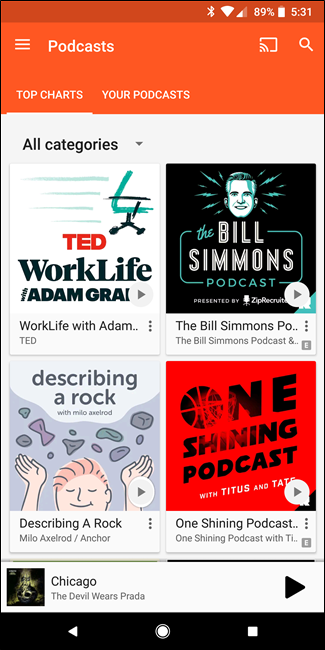In the image, an iPhone is open to a podcast app, displaying a vibrant and organized interface. The top of the screen features an orange-colored bar showing a full WiFi signal, an 89% battery level, and the current time, 5:31. Below this bar are buttons for "Podcasts," "Cast," "Search," "Top Charts," and "Your Podcasts," indicating user navigational options.

The screen is currently viewing the "All Categories" section, presenting four featured podcast thumbnails. Each podcast is visually striking with unique and engaging artwork. The displayed podcasts include:
1. "WorkLife with Adam Grant" by TED.
2. "The Bill Simmons Podcast."
3. "Disgraceland" with host Jake Brennan.
4. "One Shining Podcast" with Titus and Tate.

At the bottom of the screen, a playback bar reveals the current audio playing: "Chicago" by The Devil Wears Prada, suggesting the user is actively listening to music. The overall design is functional and visually appealing, making it easy for users to navigate and discover new podcasts.